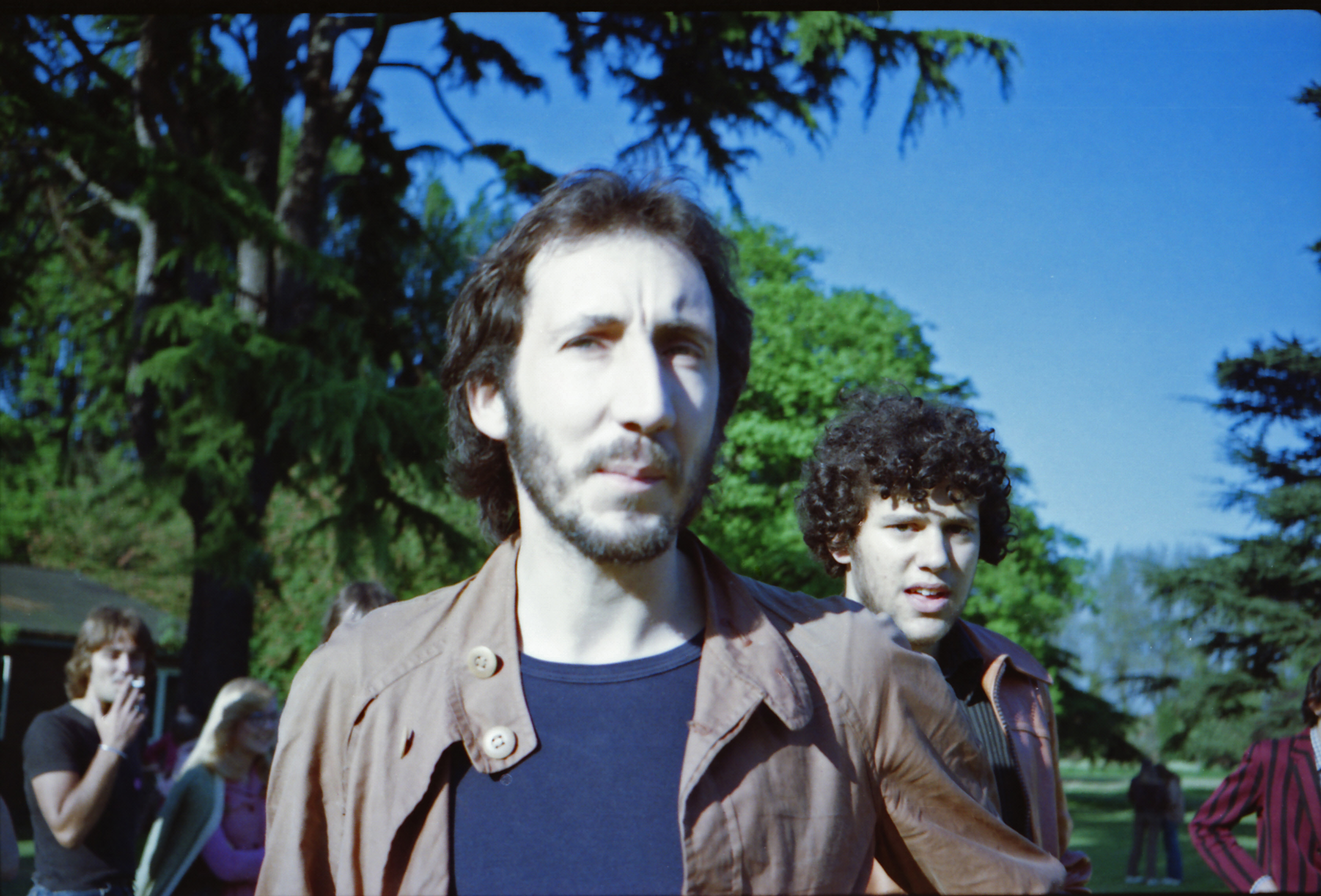In this outdoor mid-day photograph, a group of people stands in a sunlit, open grassy field against a backdrop of green trees. The central figure, a man, has short dark hair, facial stubble, and wears a thin brown jacket over a blue shirt. He appears focused or pensive. Directly behind him stands another man with very long, curly hair, squinting slightly. Further in the background, several other individuals are visible, including a woman with long blonde hair and a man smoking in a dark short-sleeved shirt. Additionally, a person wearing a dark and red striped shirt or jacket can be seen to the left of the foreground man. The upper part of the image reveals a clear, bright blue sky, predominantly in the top right corner. The photo has a blue hue and no text. The color palette includes shades of black, light blue, blue, green, gray, brown, tan, red, maroon, and pink, adding to the vividness of the scene.